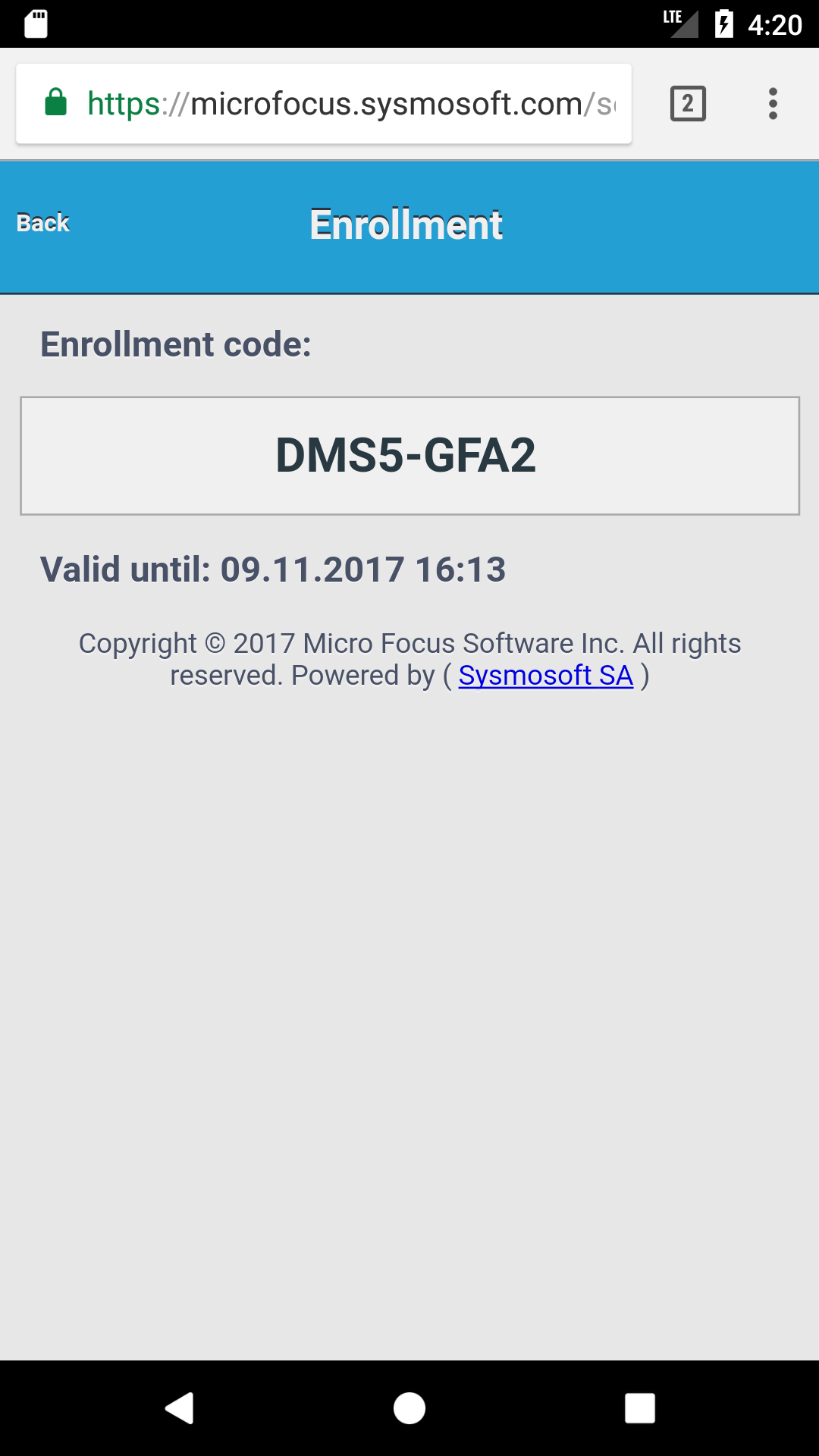The image features a smartphone screen with the following detailed elements:

- At the top is a black status bar containing various icons: a white icon resembling a gasoline barrel, LTE signal indicator, fully charged battery icon with a lightning bolt, and the time displayed as 4:20.
- Directly below the status bar is a search bar featuring a green lock icon and the URL “https://microfocus.sysmosoft.com/”. To the right of the URL box are a square icon with the number 2 in it and three vertical dots.
- Below the search bar is a section titled "Enrollment" with a blue button labeled "Back".
- Under the "Enrollment" title, there is the text "Enrollment Code:" followed by a white input box containing the code "DMS5-GFA", which is written in all caps.
- Further down, the text "Valid until 09.11.2017 16:13" is displayed, indicating the expiration date and time.
- Beneath this, the text “© 2017 Micro Focus Software Inc. All rights reserved.” is shown, along with “Powered by Sysmosoft SA” underlined and with underscores.
- The entire content rests on a gray background, and at the bottom of the screen is another black bar with phone navigation buttons: a back arrow, a home circle, and a multitasking square.

This detailed caption describes each element of the phone screen comprehensively, providing a clear visual of the image.